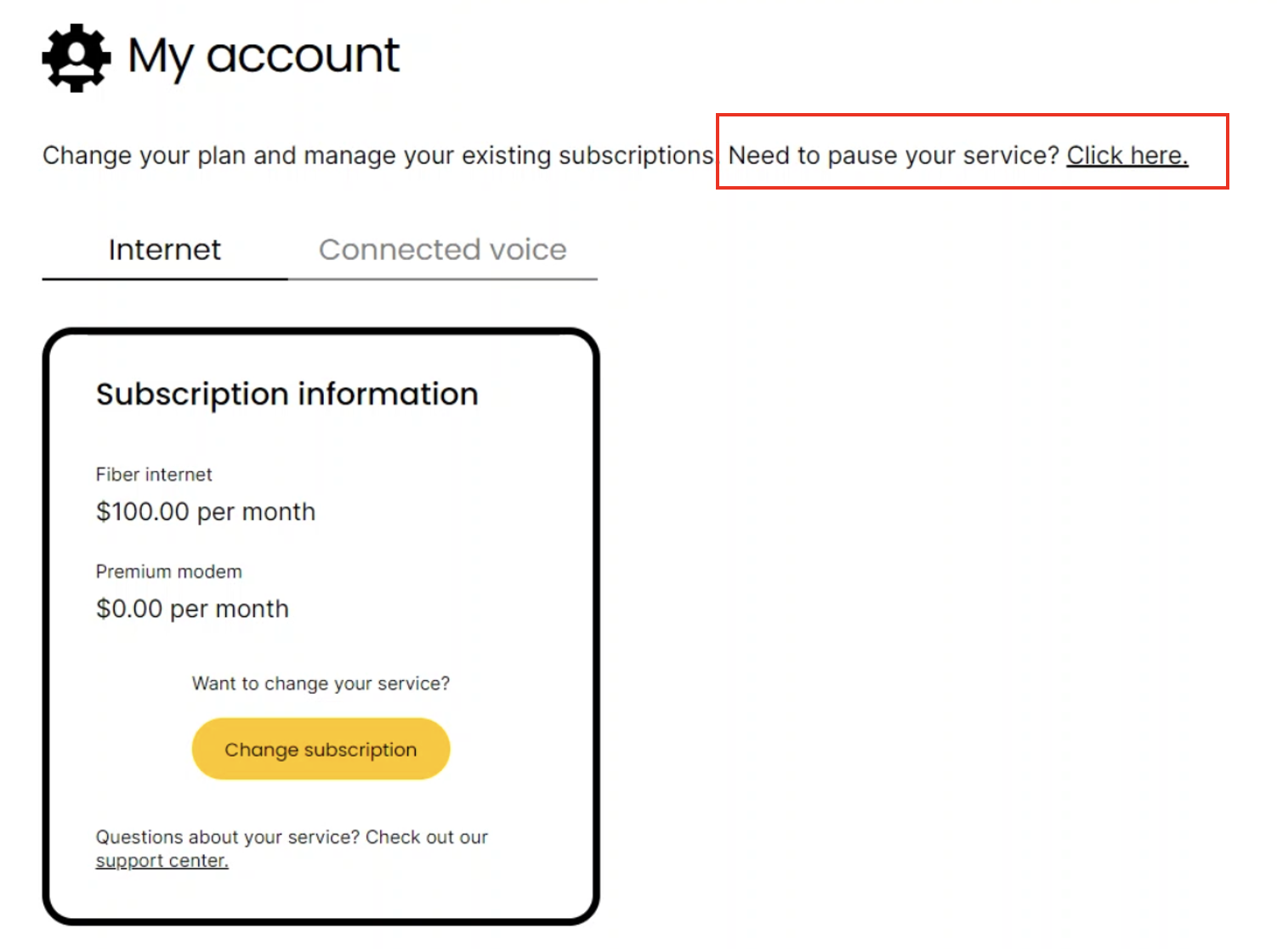Screenshot of a desktop web page featuring a section from the user's account management area. The background is predominantly white. At the top left corner, there is a heading that reads "My Account." Adjacent to it is an icon of a black gear with eight cogs, containing a white user icon inside. 

Below this, in black text, it says, "Change your plan and manage your existing subscriptions." To the right, in a red rectangle with underlined text, it reads, "Need to pause your service? Click here."

Further down, on the left-hand side, there are menu options with "Internet and Connected Voice" listed, and "Internet" is currently in bold, indicating it is the selected option.

Directly below, there is a box with slightly rounded edges and a black border. The header in the box states, "Subscription Information" in bold black text. This section details the user's current plan: "Fiber Internet, $100 per month," followed by "Premium Modem, $0.00 per month." There is an option underneath that says, "Want to change your service?" which is accompanied by a yellow button labeled "Change Subscription."

At the very bottom of the section, it reads, "Questions about your service? Check out our Support Center," with "Support Center" highlighted as a clickable link.